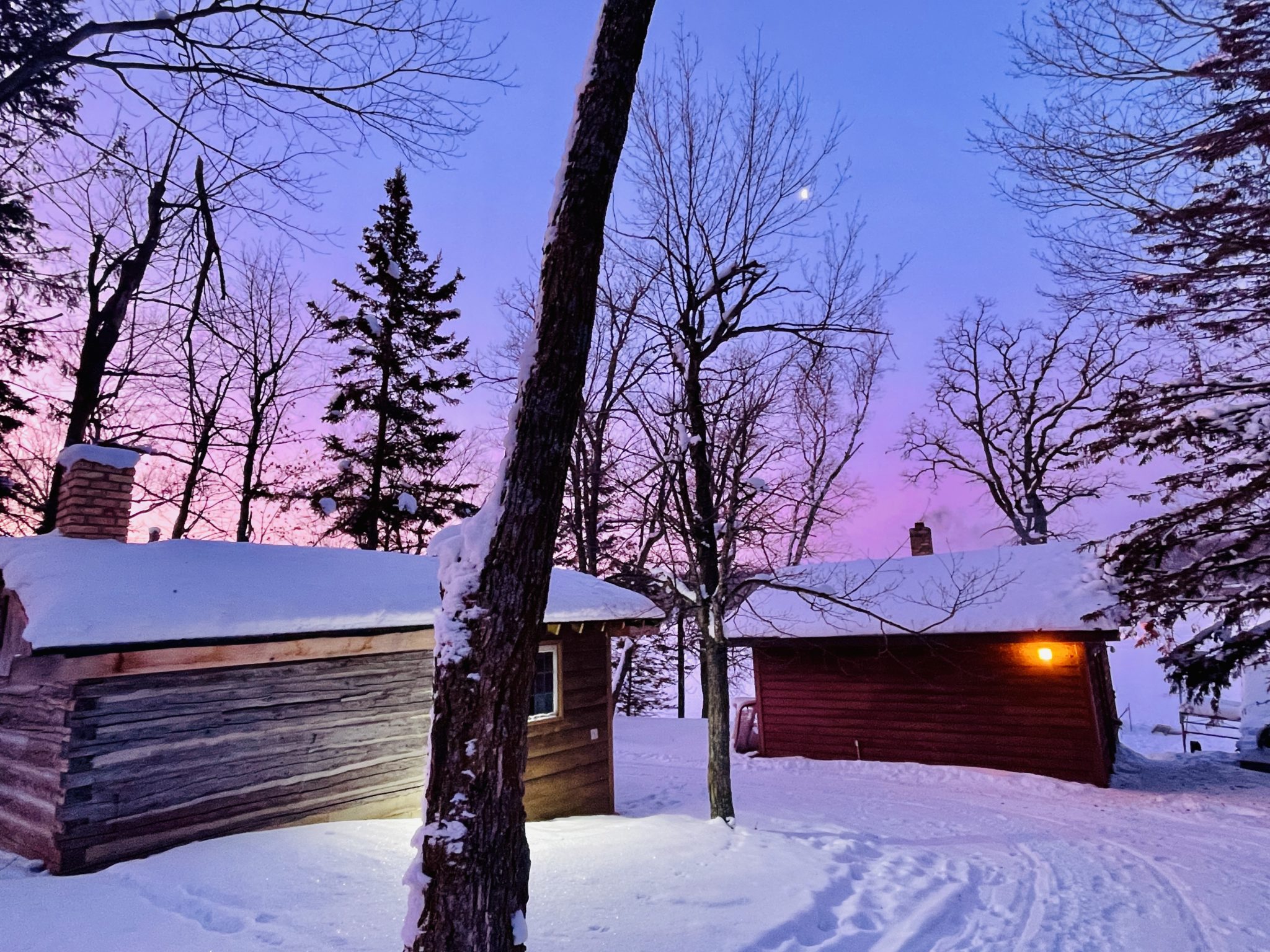The photograph captures a serene winter landscape at dusk, featuring two log cabins nestled in freshly fallen snow. The sunset casts a purplish hue near the horizon, which gradually transitions into a deep blue sky overhead. A faint moon can be seen above. In the foreground, snowmobile tracks curve around a large barren tree on the left, stretching across the snow-covered ground. To the right of these tracks stands a small red-painted log cabin with a red brick chimney emitting a curl of smoke, warmly lit by an amber light affixed to its side. Across the path, there's a larger, naturally brown log cabin also topped with snow and a brick chimney. The scene is dotted with a mix of barren trees and a few verdant fir trees, enhancing the tranquil, rustic ambiance.